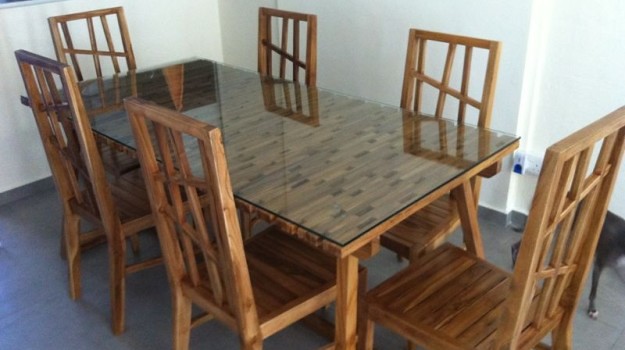This detailed image showcases a wooden dining room table with a removable glass top, set in a room with white walls and a blue carpeted floor. The table is rectangular and is accompanied by six rustic wooden chairs, three on either side and one at each end. All the chairs, matching in material and style to the table, lack cushioning but reflect a robust, natural charm. Although the room appears minimally furnished, there is a faint glimpse of another table behind one of the chairs. Additionally, a possible presence of a dog partially hidden by a chair suggests a homey atmosphere. The quality of both the table and chairs looks high, making it a potential listing for sale on platforms like Craigslist or Facebook Marketplace.